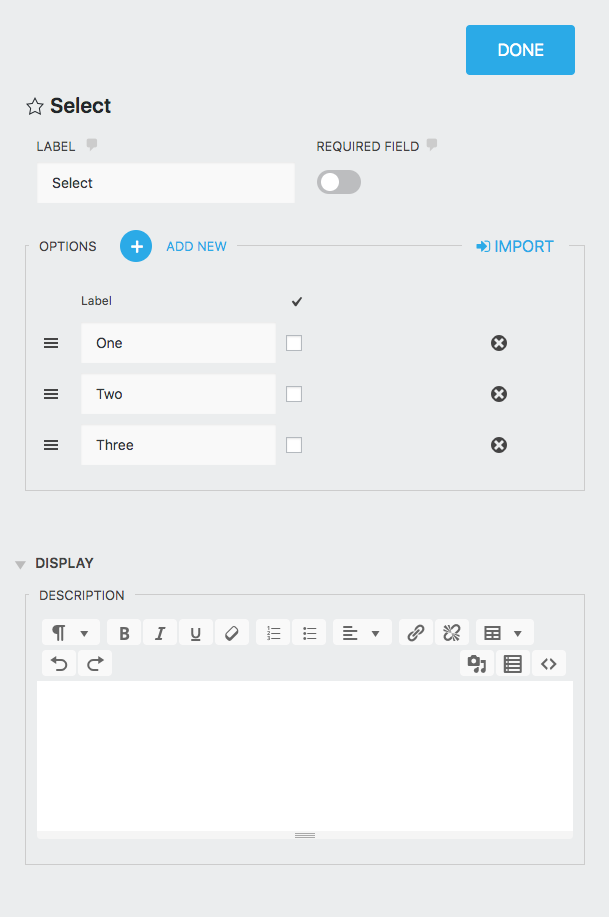This screenshot showcases a pop-up menu from a website or app, displayed against a light gray background. 

### Top Section:
- **Upper Right Corner:** There is a light blue square with the word "Done" written in white.
- **Upper Left Corner:** Features a five-pointed star icon next to the word "Select" in bold black font.

### Middle Section:
- **Field Label:** Beneath "Select", there is a text field with the placeholder "Select". Above this field, it says "Label" in black font.
- **Required Field Toggle:** To the right of this field, there is "Required Field" text with an accompanying toggle switch beneath it, currently toggled off.

### Options Section:
- **Options Header:** Below the toggle switch, a rectangle is labeled "Options". 
- **Add New Option:** To the right of this header, there is a blue circle with a white plus sign, followed by the text "Add New" in blue font.
- **Import Option:** Further to the right, there is a share icon accompanied by the text "Import".

### Checkable Fields:
- **Label and Fields:** Below the "Options" section, it says "Label" in black font. There are three text fields underneath, each with a corresponding checkbox.
  - The fields are numbered "1", "2", and "3".
  - To the right of each field, there is a black circle with a white "X" in it.

### Display Section:
- **Display Header:** There is another rectangle labeled "Display".
- **Description Field:** Below "Display", it says "Description", followed by a large white text field where users can enter text.